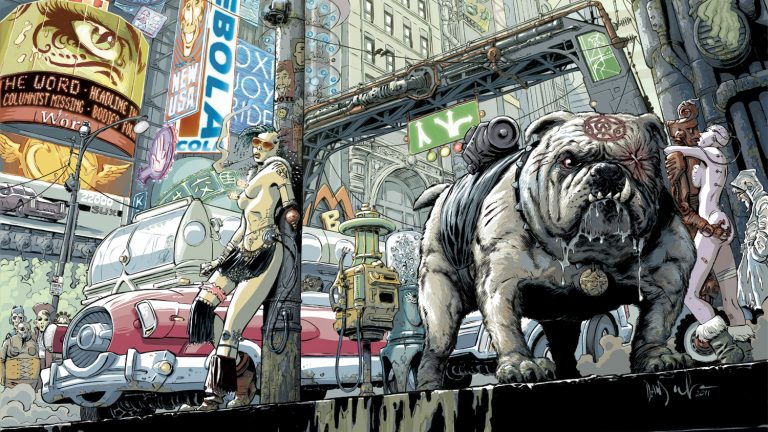This illustrated scene from a comic book depicts a bustling post-apocalyptic cityscape. The background is filled with tall, gray skyscrapers adorned with a variety of neon billboards, contributing to the chaotic yet vibrant atmosphere. Notable signs include a green-skinned eyeball billboard with a headline reading, "The Word: Headline, Columnist Missing, Bodies Found," as well as ads for "Bola Cola," "New USA," and a partially obscured blue advertisement for "Oxi Oi Ride." An overpass constructed from metal tubes stretches across the street, with a green sign dangling from it, featuring two sets of white arrows. Beneath the overpass, a scene unfolds at street level with a red vehicle and a beige bus featuring large front windows.

Central to the scene, leaning against a tall utility pole, is a striking woman. She wears a black loincloth and fringed boots, is topless but adorned with two light bulbs on her breasts, and accessorized with red-tinted sunglasses. Her blue dreadlocks cascade to the side, and her left arm is replaced with a brass ball. To the right, a gray pit bull stands solemnly. It bears a red five-pointed star tattoo inside a circle on its forehead, with its right eye sewn shut by two strings. The dog is draped in black fabric, upon which rests a gray gun. The surreal, hand-drawn cityscape exudes a distinctive post-apocalyptic vibe, blending elements of urban decay with futuristic and dystopian visuals.